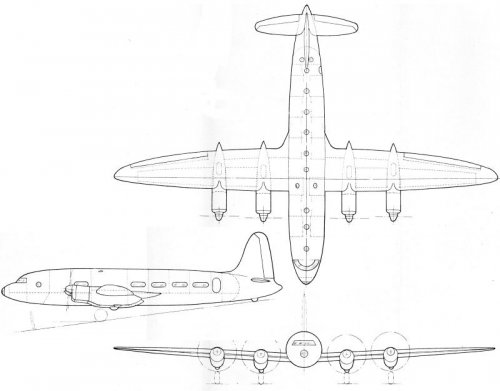This detailed, black-and-white blueprint-style sketch of an airplane features three distinct views of the aircraft. The top image provides an overhead perspective, displaying the expansive wingspan extending from left to right, the body of the airplane with its nose oriented at the bottom, the tail at the top, and the windshield toward the aircraft's front. The left-side drawing shows a side profile with notable details such as four windows along the fuselage, a prominent cockpit at the front, a door positioned toward the tail end, and one of the aircraft's wings. Finally, the bottom sketch captures a front-facing view of the plane, highlighting its four rotor-driven engines—two on each wing—flanking the cockpit, with the tail visible in the distance. The entire composition is rendered meticulously on what resembles graphing paper, emphasizing the technical precision of the design.